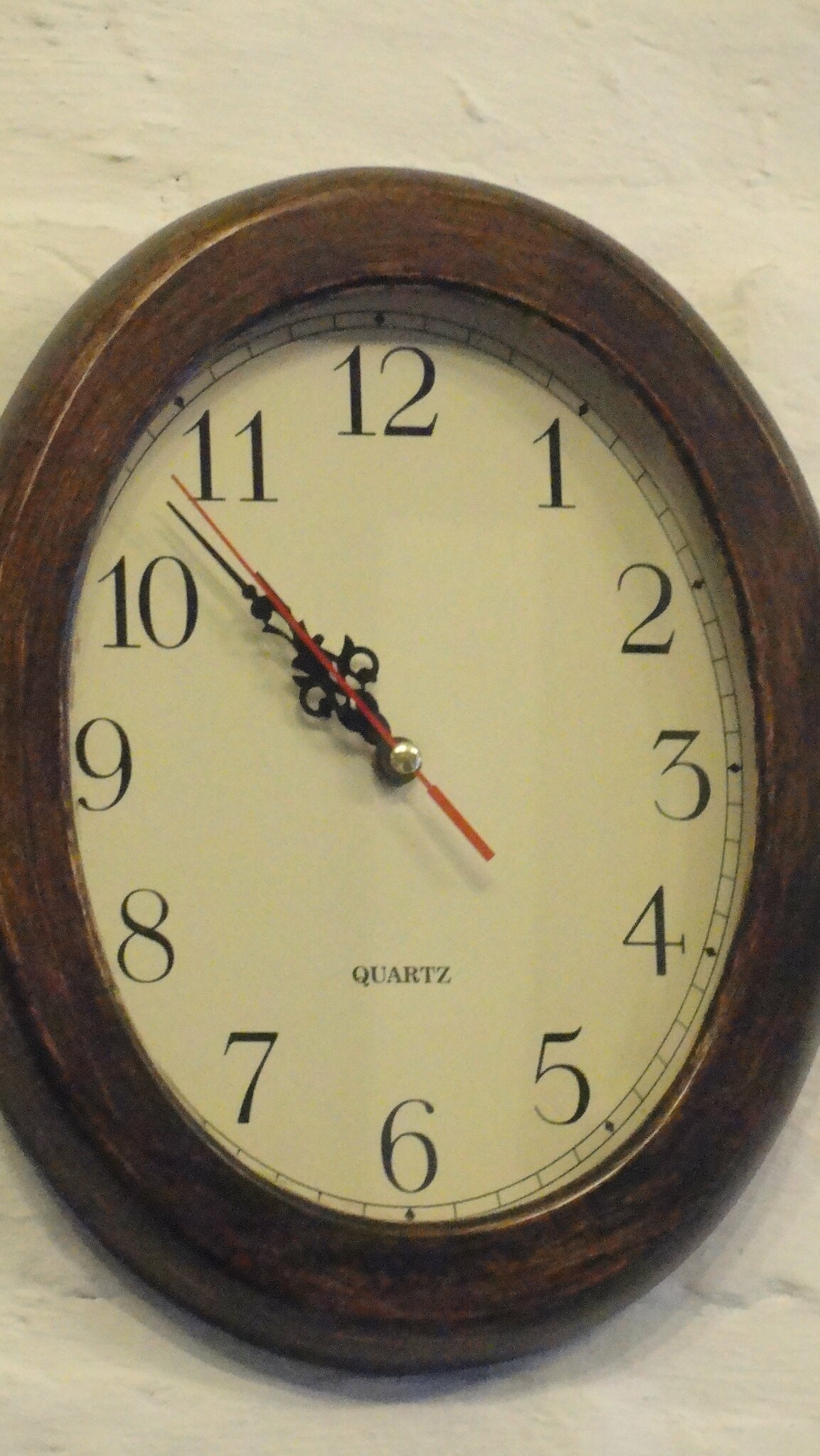In the foreground, there is a grand clock encased in a rich brown wooden frame. The frame has intricately carved edges that protrude slightly, giving it a distinctive, ornate look. The clock face is predominantly white and features black numerals ranging from 1 to 12, positioned around the perimeter. Surrounding the numerals, dark dots are situated at each hour mark, complemented by smaller dashes forming squares and rectangles along the outer edge. The center of the clock showcases the minute, hour, and second hands, all aligned and pointing between the 10 and 11 o'clock positions. The clock face is subtly recessed into the wooden frame, adding depth to its design. In the background, a white stone surface adds a contrasting backdrop to the warm wooden tones of the clock, though the details of the stone are indistinct.